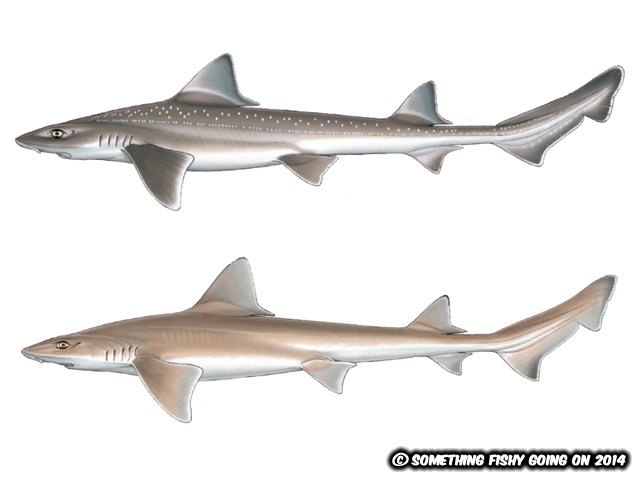The image features two computer-generated illustrations of slender, elongated fish, likely sharks, set against a solid white background. The sharks are positioned one above the other, both facing left. The upper shark is dark grayish-brown with a silvery-white underside and adorned with small white dots along its back. The lower shark, similar in shape and size, displays a lighter brown top with a corresponding light gray underbelly. Each shark has long, streamlined bodies characterized by dorsal fins, side fins, and a tail fin that is more elongated at the top but splits into two smaller fins at the bottom. A distinguishing copyright notice is present in the lower right corner of the image, in white text with a black shadow, reading "Something Fishy Going On 2014".